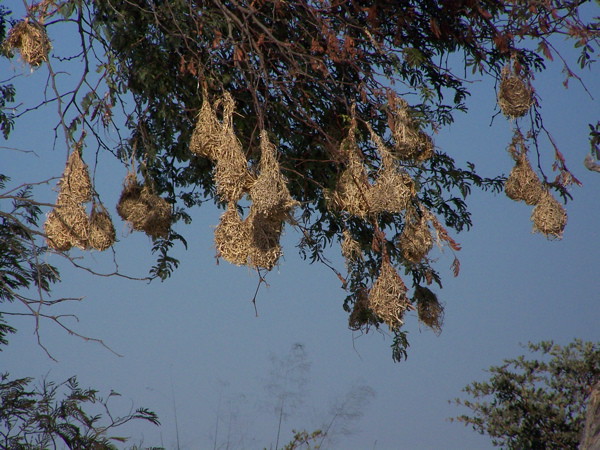This photograph, taken on a bright day with a blue sky, features a close-up view from beneath a tree, capturing both its green and dead leaves. The main focus is the tree, which resembles a fern or conifer, showcasing a mix of vibrant green leaves and peculiar gray, dead leaves that almost look like bats hanging from the branches. Additional oddities include light brown, hay-colored objects, resembling upside-down straw birds' nests, hanging from the branches. In the distance, the tops of other trees are visible, framing the main subject and adding depth to the outdoor scene. The image quality is not the best, but the details are still discernible, evoking a sense of fall.